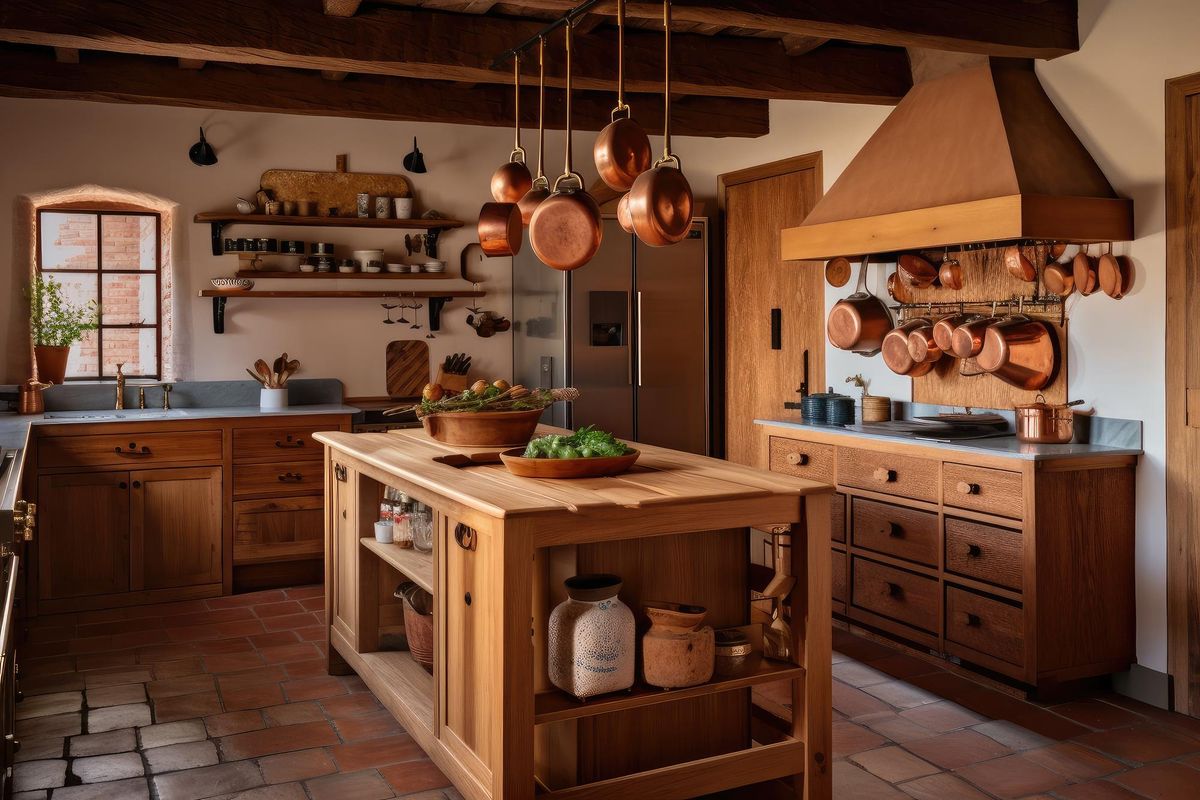This image portrays a rustic-style kitchen bathed in morning light, evoking the charm of an old-fashioned house. The room features a cobblestone tile floor and off-white walls adorned with numerous copper pots, lending it a warm and inviting ambiance. Prominent among the fixtures is a large hooded vent with several hanging copper pots, enhancing the kitchen's earthy aesthetic. The wooden island at the center stands out, storing cooking utensils and supplies, and its countertop displays a bowl of green vegetables and another bowl with stalks.

The drawers and cabinets are crafted from rich wood, complemented by a greyish-blue countertop that adds contrast to the otherwise warm hues. Sparse counter space hosts a utensil jar, while two shelves on the wall hold various jars, spices, and kitchen objects, including a canister with spoons, a cutting board, and a small plant near the window. This window, situated above the sink, provides natural light and a view to the exterior.

Additional details include metal, likely bronze, pans hanging over the island on the right side, and antique jugs and cut flowers awaiting arrangement on the island's surface. The kitchen scene, possibly AI-generated but remarkably realistic, captures a blend of utility and rustic charm, showcasing an interplay of textures and colors that invite a homely atmosphere.